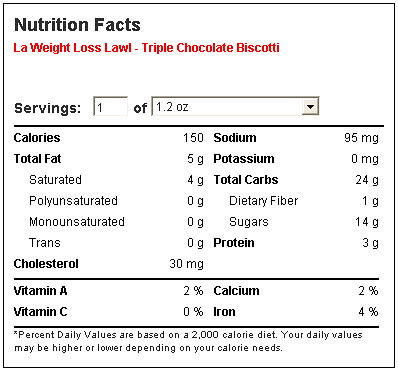On a stark white background, a detailed white nutritional label features prominently. The label includes black text stating "Nutritional Facts" and a bold red banner that reads "LA Weight Loss" followed by "Triple Chocolate Biscotti." The serving size is listed as one 1.2-ounce biscotti. It specifies that there are 150 calories per serving, with 5 grams of total fat, including 4 grams of saturated fat, 30 milligrams of cholesterol, and 95 milligrams of sodium. Additionally, the biscotti contains 24 grams of total carbohydrates, including 14 grams of sugars, and 3 grams of protein. The label also notes the presence of essential nutrients: Vitamin A, Vitamin C, calcium, and iron. The percentages for these values are based on a 2,000 calorie diet.